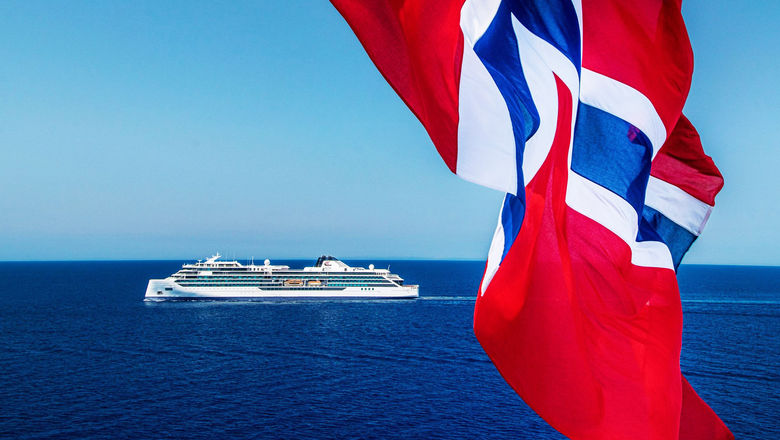The image depicts a massive white cruise ship with multiple levels and numerous windows, sailing across a strikingly deep, velvety blue ocean. The sky above is a contrasting light blue, clear and cloudless, creating a clean, distinct horizon line. The water, unusually rich and dark, mirrors the intense blue hue present in both the sea and the background, making the ocean almost resemble velvet. The cruise ship, positioned toward the left of the photo, appears to be moving from right to left, indicated by the visible trail of white wake behind it. In the foreground, a red, white, and blue flag flutters in the wind, though its exact design and origin remain indeterminate. The flag's vibrant colors, particularly the deep blue, harmonize with the maritime scene, further enhancing the natural splendor and vividness of the photograph.